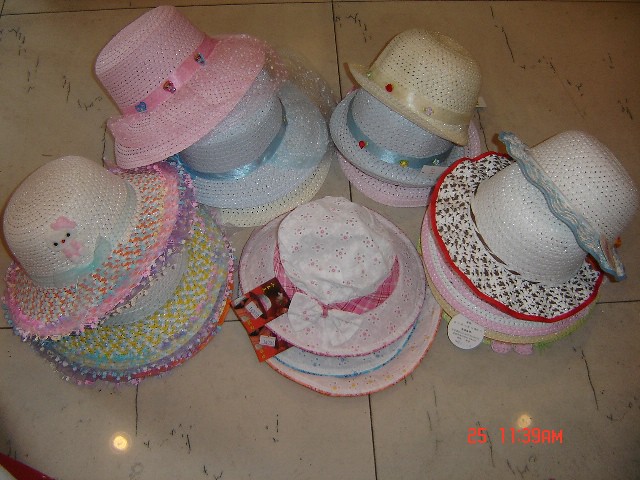The image captures an assortment of children's hats arranged in multiple stacks on a white marble countertop with black streaks and blotches. Each stack showcases hats with a woven texture, resembling plastic or synthetic fibers, adorned with various colorful decorations. The prominent hat features a small standing cat with black eyes, a red nose, a pink bow, and a pink shirt, intricately embroidered in pink, red, blue, white, and purple threads. Another hat is primarily blue with gold, light blue, cyan, and purple stitching. Other noticeable hats include ones with purple frills or red accents, and several feature flower embroidery in pink. The pink and white hat at the top has a red and maroon plaid ribbon with white stripes, while those beneath are blue and orange. A nearby stack includes a pink hat with a matching ribbon adorned with faint hearts and shapes, a similar blue hat, and a tan one. Another stack follows with tan hats embellished with green, red, and purple flowers on a tan ribbon, a blue hat, and an obscured pink hat. A final set of hats includes a white hat with floral embroidery and a blue rim, a white hat with chocolate brown and white snowflake-like designs, a hot pink and white-striped hat, and a concealed tan hat. The scene is timestamped in red text at the bottom right, indicating the photograph was taken at 11:39 a.m. on the 25th.